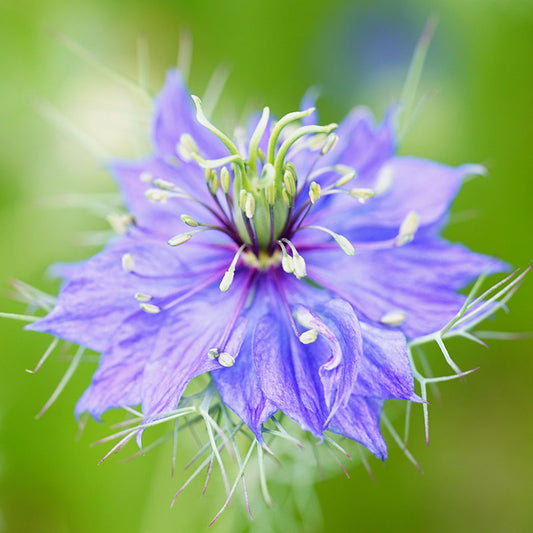This macro close-up photograph features a vibrant purple wildflower with a unique and intricate petal arrangement resembling a star with over a dozen spear-shaped petals. The flower's petals protrude in various directions, forming a complex and non-symmetrical pattern. The center of the flower showcases a green plumage with numerous thin, spiky tendrils, each tipped with a small bright green seed pod. Some tendrils have a distinctive purple stem. Surrounding the central area are Y-shaped green branches with purple tips, adding to the flower’s detailed texture. The background is a vivid, blurred green, highlighting the flower's striking features and drawing focus entirely to its elaborate structure.